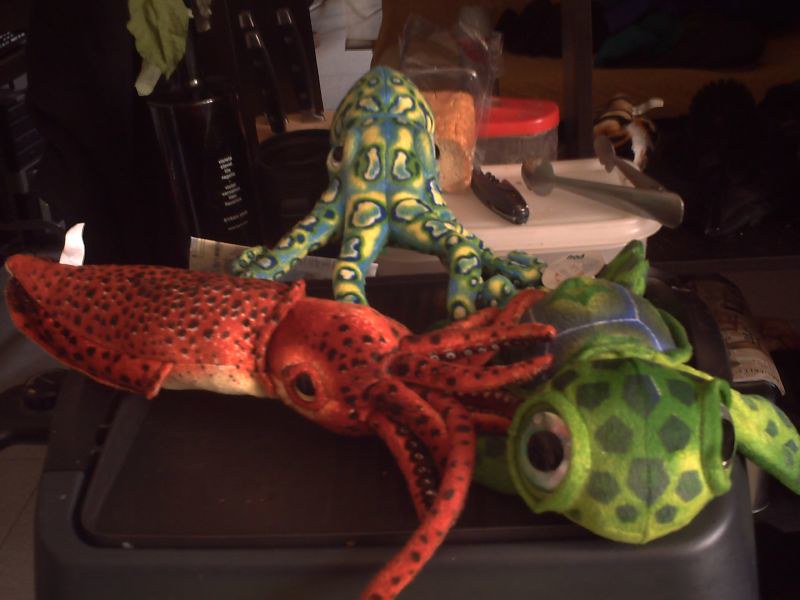This indoor photograph is quite dark, making the background elements hard to discern. In the foreground, three stuffed sea animals are prominently displayed atop a black plastic wastebasket or carrier. On the left side is a red stuffed shrimp or squid adorned with white and black dots. Beside it, in the center, is a vibrant blue and yellow octopus with swirling colors and patches resembling a dye pattern. On the right side occupies a light green and yellow turtle with distinctive green spots. Further into the blurred background appears a clear container with a white lid, possibly Tupperware, with what seems to be a metal spoon resting on top, alongside what might be a wine bottle. The setting suggests a dining room table.